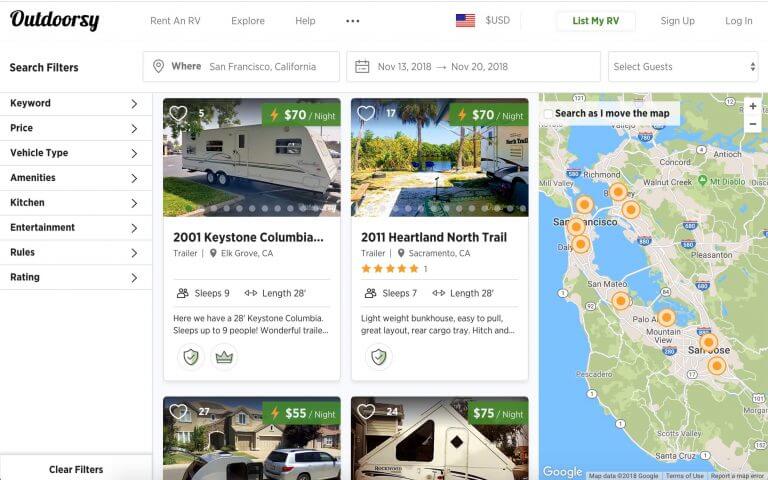This is a detailed photo of the Outdoorsy website interface. In the upper left-hand corner, the word "Outdoorsy" is prominently displayed in black, uppercase letters. Adjacent to the right is a white search bar, followed by a horizontal menu with grey font options: "Rent an RV," "Explore," and "Help," alongside three additional menu buttons. Continuing to the right, there is a space leading to icons for currency selection, featuring an American flag and a dollar sign indicating USD.

Further to the right, you'll find the "List My RV" button, as well as "Sign Up" and "Login" buttons, neatly aligned at the top. Directly beneath the "Outdoorsy" logo on the left-hand side, there's a vertical navigation menu.

Dominating the main window to the right of this vertical menu are four distinct blocks, each showcasing an RV; these are arranged in a 2x2 grid format, with two blocks on the top row and two on the bottom. On the right-hand side of the page, there is an interactive map with a label that prompts users to "Search" or "Move the Map" to refine their RV search criteria and explore different locations.